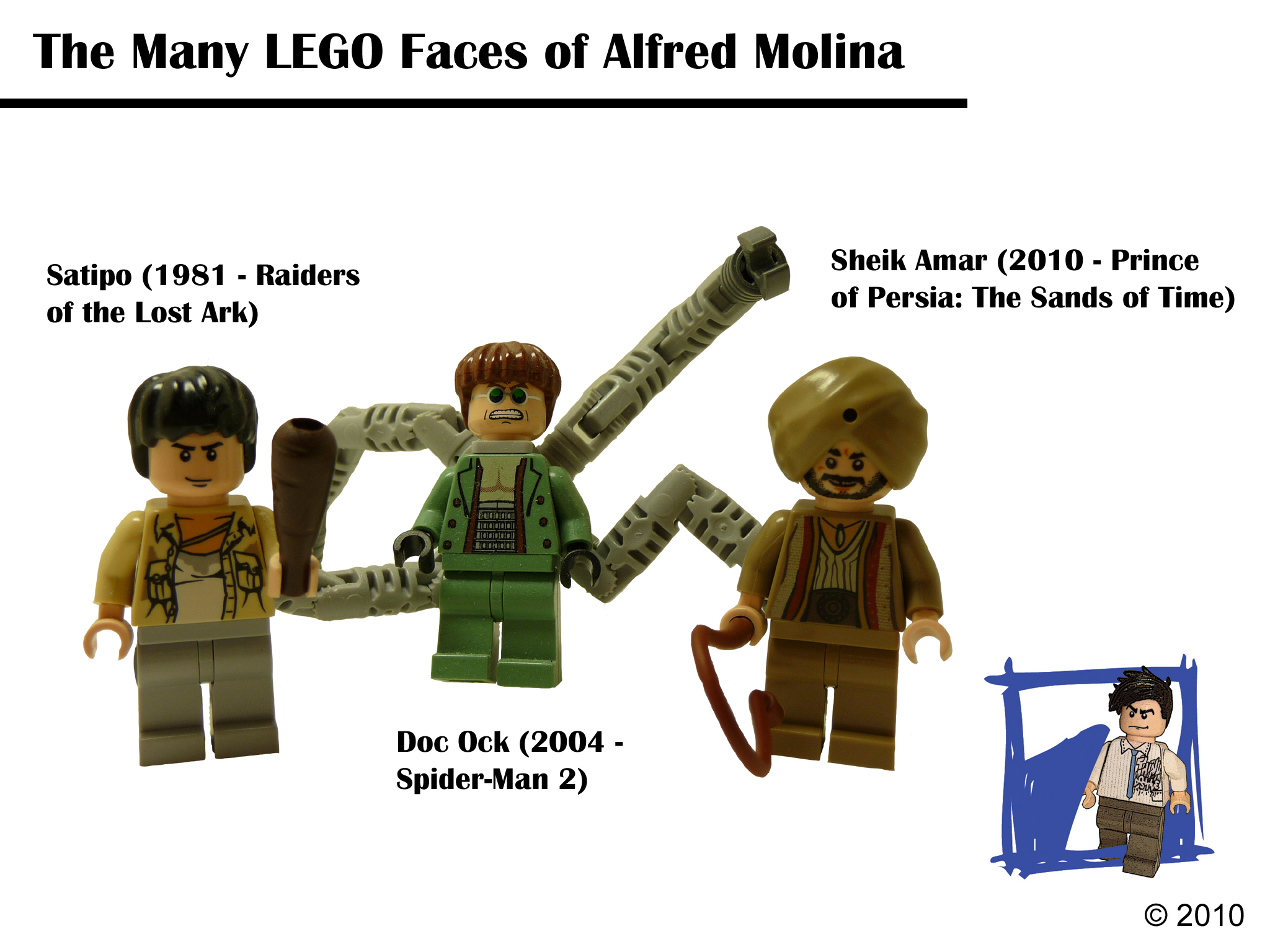This image, titled "The Many Lego Faces of Alfred Molina," features four detailed Lego minifigure representations of characters portrayed by the actor Alfred Molina. In bold black letters beneath an underline, the title points out the diverse roles Molina has played. Each minifigure is meticulously labeled with the character's name, year, and associated movie:

1. The first minifigure depicts Satipo from "1981 Raiders of the Lost Ark," dressed in a yellow top and gray pants, holding a wooden club.
   
2. The second minifigure portrays Doc Ock from "2004 Spider-Man 2," characterized by a green suit, glasses, and the iconic multiple mechanical arms extending from his back.

3. The third minifigure represents Sheikh Amar from "2010 Prince of Persia: The Sands of Time," wearing a turban and carrying what appears to be a shepherd's crook or whip.

4. Embedded in the image's bottom right is an additional illustration of Alfred Molina’s Lego form wearing a white sweater, brown pants, and a blue tie.

At the lower edge, the artwork is marked with a copyright note from 2010.